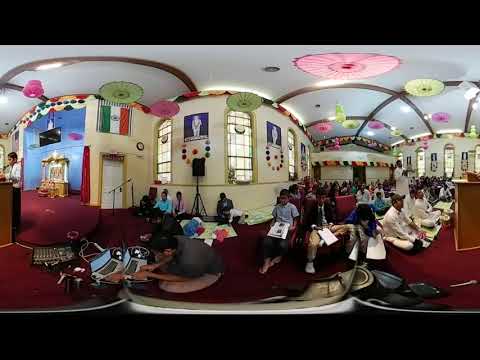The image depicts an indoor event space, possibly a church or a school building, that has been elaborately decorated for a ceremony or gathering. The photo is a 360-degree shot, resulting in significant distortion that makes it difficult to discern straight lines and the true curvature of the room. 

On the upper left side of the image, there's a person standing on a podium speaking into a microphone, with another podium on the right side that might be connected due to the distortion. Behind the speaker, a large blue backdrop is visible, featuring a golden statue or display. A cream-colored wall runs along the length of the building.

Across the room, numerous decorations adorn both the walls and the ceiling, including colored fans in yellow and pink, as well as various discs. A prominent black horizontal element, possibly a wall or barrier, spans the lower part of the photo. 

A significant crowd, comprising both adults and children, is seated on the floor, many in white uniforms and some in a lotus position. A person in the bottom left corner is working on a laptop. The right side of the image shows another group of people seated on the floor, with one individual standing amongst them, appearing to be looking towards the right. The overall scene is lively with various art pieces and colorful decorations, suggesting a celebratory or communal event.